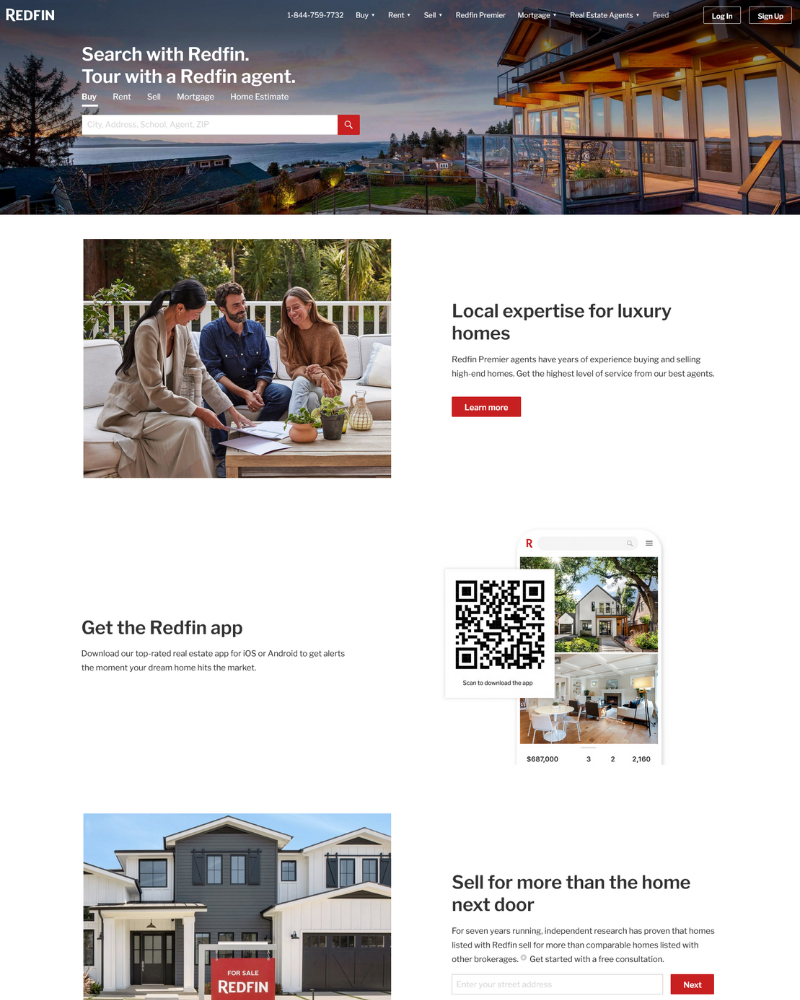This is a detailed descriptive caption for the provided image:

#### Descriptive Caption:
The screenshot showcases the Redfin website's homepage, adorned with a vibrant header image capturing a serene environment with blue skies, an ocean on the left, and lush greenery. To the right, a quaint log cabin with an expansive deck stands prominently, while in the distant background, additional houses and trees are visible, enhancing the picturesque setting.

In the top-left corner of the header, the Redfin logo is displayed in white. Adjacent to this, a contact number is listed: 1-844-750-7732. Sequentially to the right, a navigation menu includes the following options, each accompanied by a downward-facing arrow: "Buy," "Rent," "Sell," "Book a Property," and "Mortgage." The menu extends further with two unreadable options, concluding with a "Login" button and another blurred button.

Beneath the header image, on the left-hand side, a smaller photograph features three individuals seated on a couch. The group consists of a woman with dark hair in a white dress, a bearded man in a blue shirt and jeans, and another woman with brown hair dressed in a brown sweatshirt and blue jeans. To the right of this photo, black text reads: "Local expertise for luxury homes." Below this, additional text is too blurry to decipher, with a prominent red "Learn More" button visible.

Moving further down the page, bold text on the left declares: "Get the Redfin app," though the accompanying description is unreadable. Adjacent to this, a conspicuous QR code is displayed, flanked by two thumbnail images. The upper thumbnail depicts the front of a pristine white house, and the lower one shows the interior of a living room and dining room combination.

At the bottom left, another large image features an elegant gray and white house, with a "For Sale" sign from Redfin presented in white letters on a red and black background. Next to this, the text "Sell for more than home next door" appears in bold black letters. An unreadable description lies beneath, with a "Next" button outlined in white text against a red background on the far right.